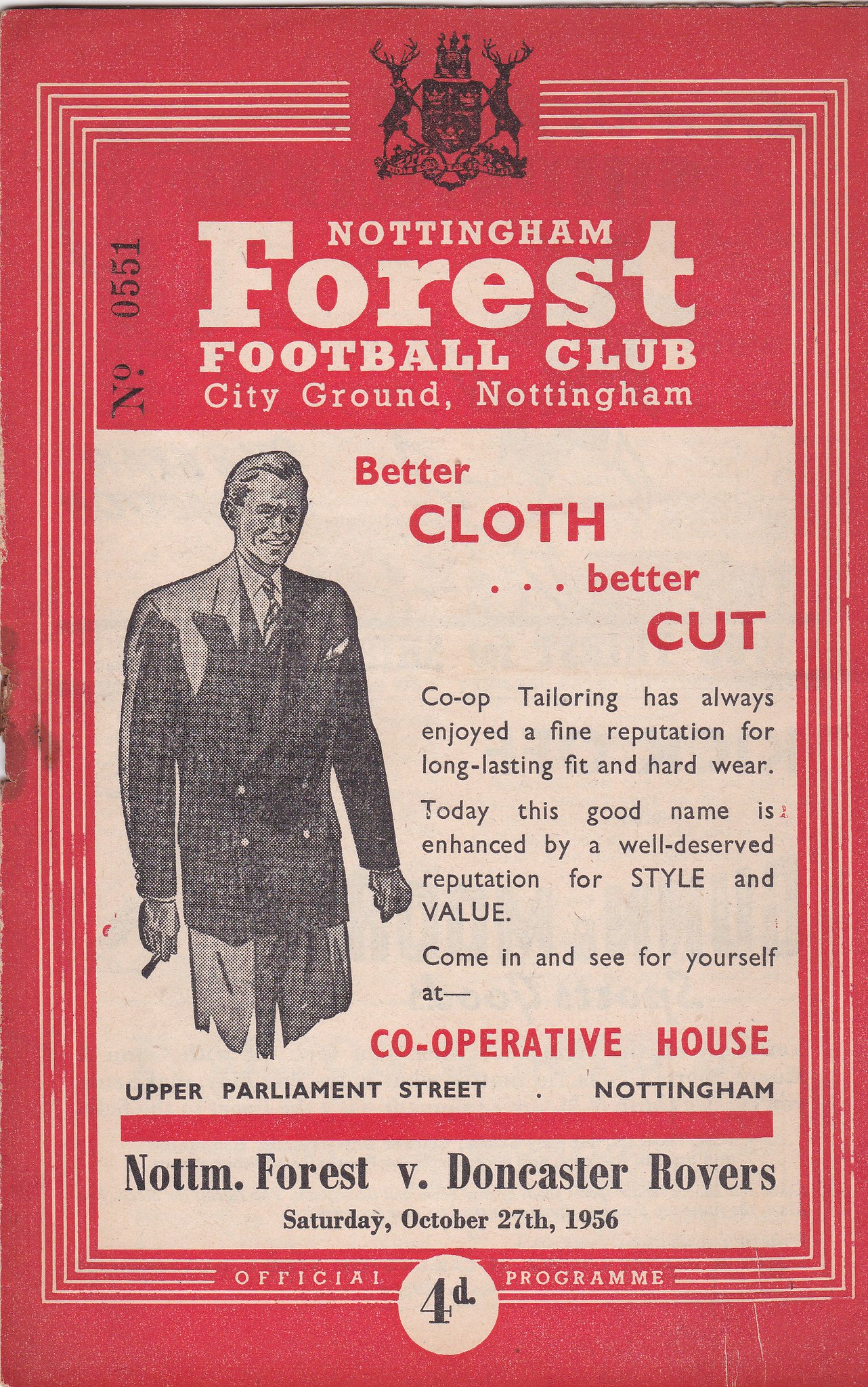This vintage 1956 advertisement for the Nottingham Forest Football Club features an official program. Against a red background, the design prominently centers on a complex pattern of concentric lines forming a square. At the top, two imposing deer with tall antlers flank a black emblem. Above this, "Nottingham Forest Football Club, City Ground, Nottingham" is written in white. To the left, in black text, the number 0551 is shown. Below, a square with a white background displays a black-and-white depiction of a smiling man in a suit, holding a cigar. The caption next to him reads "Better Cloth, Better Cut" in red, followed by "Co-op Tailoring" and an endorsement of its fine reputation for long-lasting fit and hard wear. The mention of "Cooperative House, Upper Parliament Street, Nottingham" follows in red and black text respectively. A red bar runs horizontally below, marking the match details: "Nottingham Forest vs. Doncaster Rovers, Saturday, October 27, 1956." The text concludes with "Official Program" adjacent to a white circle containing "4d," indicating the price. The overall nostalgic design, with its mix of white, red, and black elements, encapsulates the era's aesthetic and highlights the football match and tailoring advertisement.